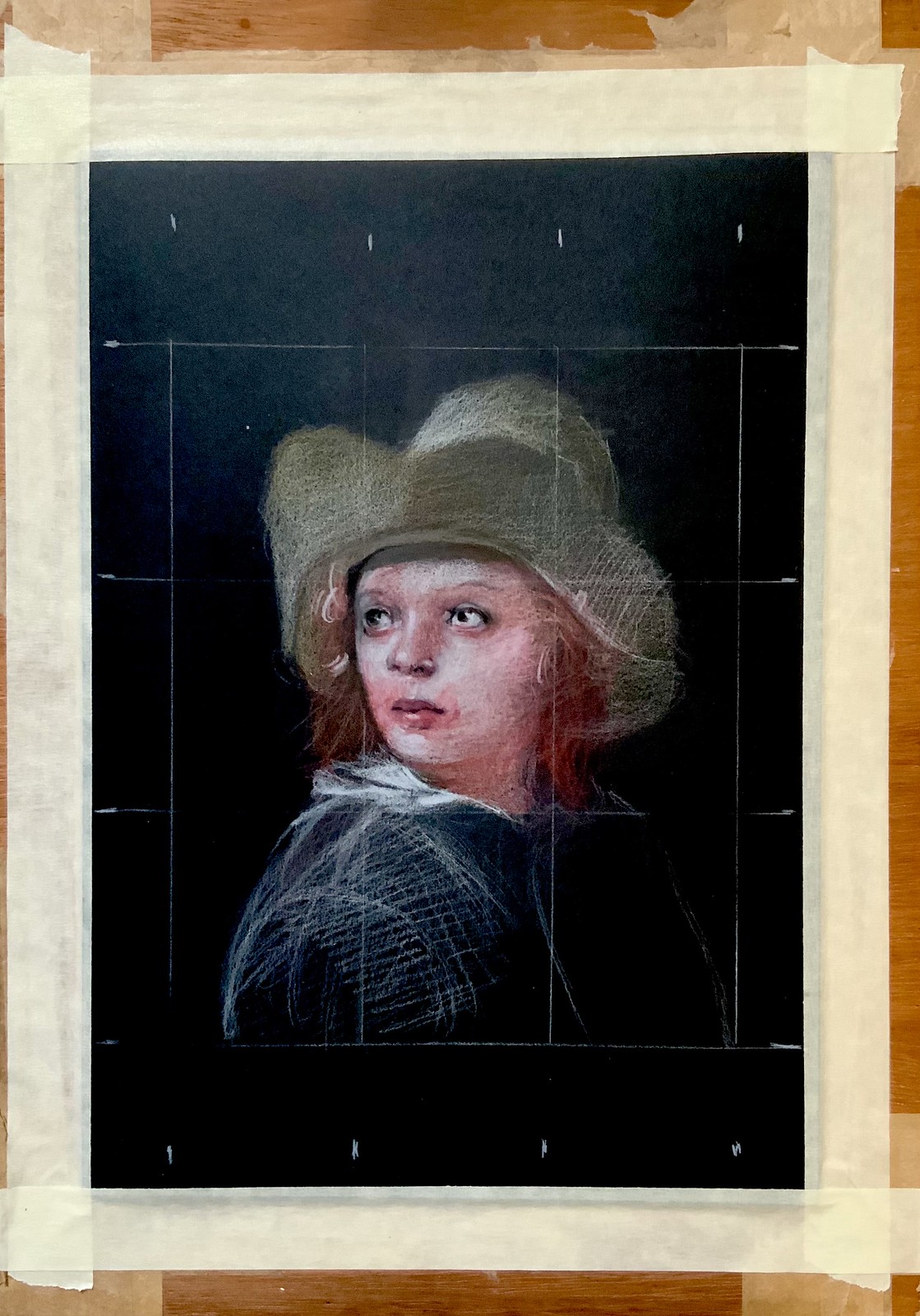This vertical color photograph captures a charcoal sketch on black paper, depicting a young boy who bears striking similarities to figures painted by Dutch masters. The boy, dressed in 16th-century attire, wears a gray-brown hat with an upturned brim, revealing his lovely reddish hair. His somber expression is accentuated as he looks over his right shoulder. He is adorned in a blackish-blue coat over a white shirt. The sketch is secured with masking tape onto a light-colored wooden board, which also has other pieces of masking tape. The background is entirely black, emphasizing the detailed lines and shading done primarily in white chalk or pencil. There is no text in the photograph, but the boy's pinkish skin tones and the exquisite attention to the textures and hues of his clothing create a vivid and captivating image.